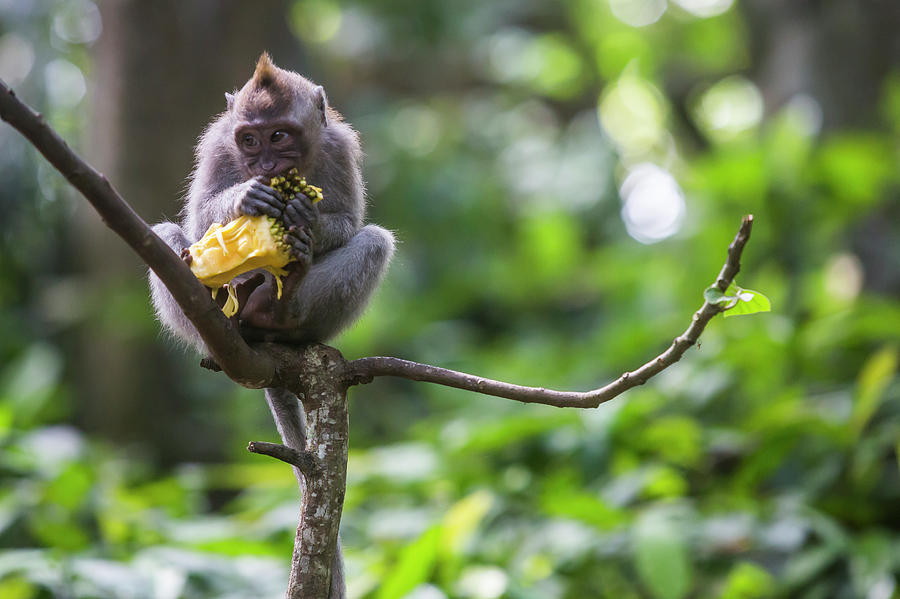In this image, the focal point is an adorable baby monkey with predominantly greyish-black fur and a distinctive tuft of brown hair on top of its head, resembling a small mohawk. The monkey is perched on a thin, forked branch, sitting comfortably in an almost crunched, Indian-style position. It appears to be in a rainforest environment, as blurred greenery forms the backdrop of the photograph, enhancing the focus on the monkey. 

The monkey is holding up a yellow fruit, possibly a type of pineapple, using both its hands and feet. The fruit, with a yellow peel and seed-like texture, is being brought towards its mouth, indicating the monkey is in the midst of eating it. The little creature’s black fingers grasp the top of the fruit, while its feet support the lower part. The image captures the moment with the monkey looking slightly to its left, intently focused on its snack. The overall scene is both charming and intimate, showcasing the monkey alone on the branch against a beautifully blurred green forest background.